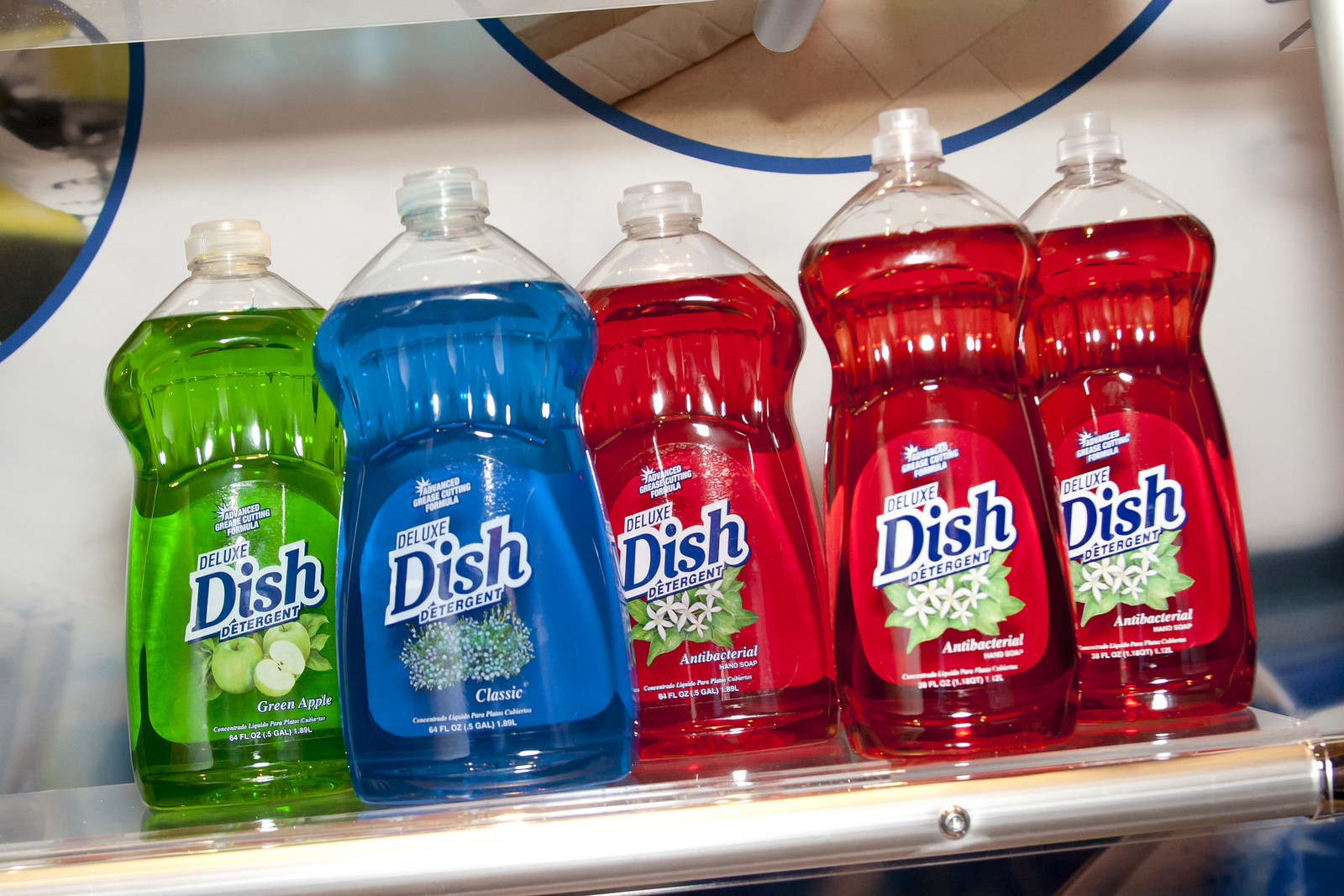The image is a bright and sharply focused close-up of several bottles of dish detergent, likely taken with a flash due to its stark contrast. The bottles are neatly lined up on a shelf, suggesting a store display. There are five bottles in total: one green, one blue, and three red. All bottles are full and have their caps intact, indicating they are brand new. The labels identify the brand as "Deluxe Dish Detergent, Advanced Grease Cutting Formula." The green bottle has an apple scent with an accompanying image of an apple, the blue one is labeled "classic" and features a floral design, and the red bottles are marked "antibacterial," each displaying a leafy plant with white flowers. Behind the bottles, there are posters, reinforcing the idea of a retail environment. The label details and the emphasized "e" in "detergent" suggest the product might originate from a Spanish-speaking country.